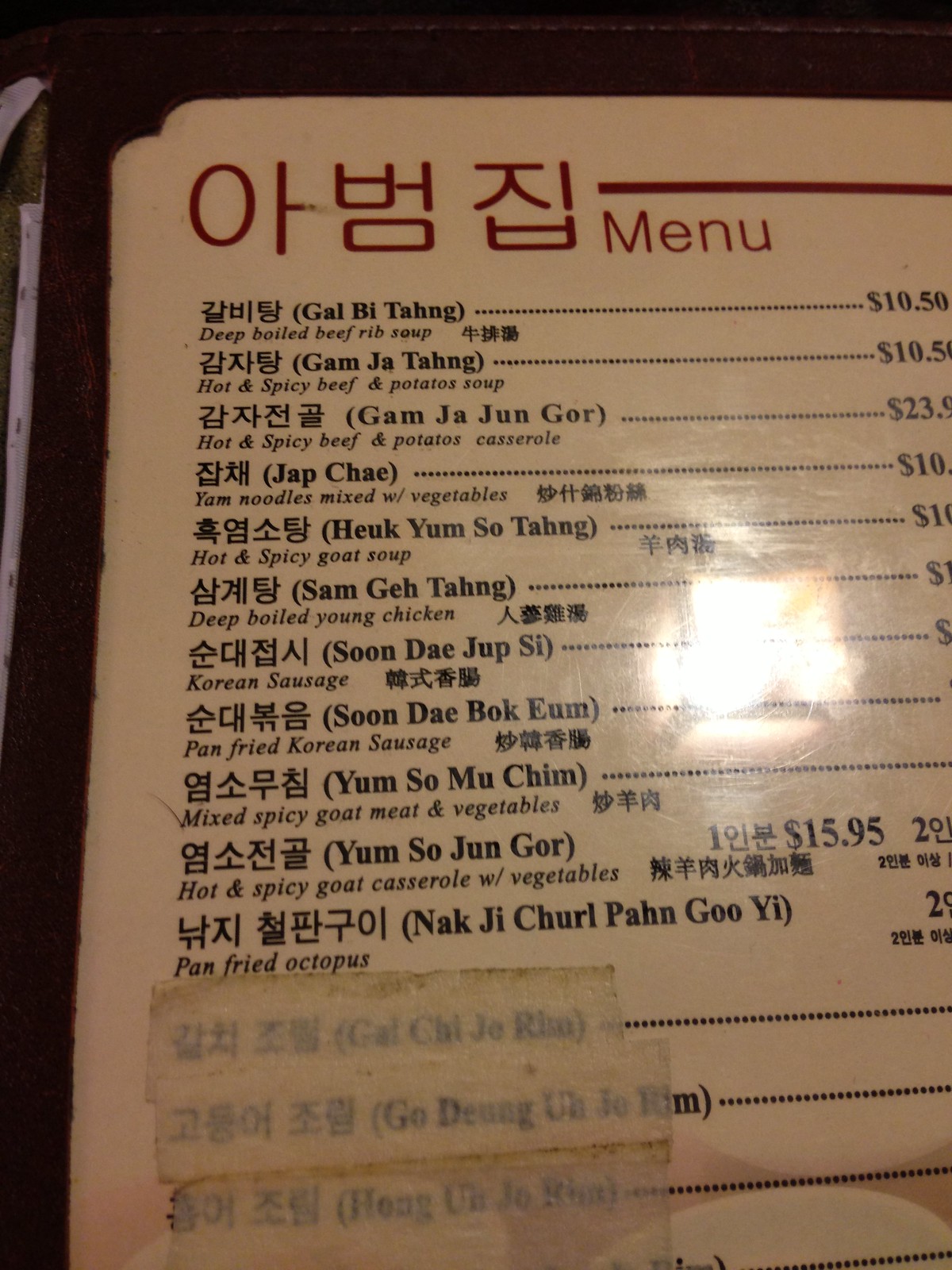This photograph displays the left side of a multi-page Korean menu. The menu is structured in a book-like format, with more than one page. At the top of the page, there is Korean text in red letters situated in the upper left corner, followed by the word "Menu" in English to the right. Below this header, approximately 15 or more menu items are listed.

Each item is featured with Korean text on the left and English translations in brackets to the right. Some of the dishes include:
- **Galbitang ($10.50)**: Deep broiled beef rib soup.
- **Gamjatang**: Hot and spicy beef and potato soup.
- **Gamja Jungor**: Hot and spicy beef and potato casserole.
- **Japchae**: A Korean dish made from sweet potato noodles.
- **Hukyumsotang**: Traditional beef soup.
- **Samgyetang**: Ginseng chicken soup.
- **Soondae Bakyum**: Stir-fried Korean blood sausage.
- **Yumsomuchim**: Spicy goat salad.
- **Yumsojungor**: Goat stew.
- **Nakjichulpan Gulbap**: Stir-fried octopus with rice.

Each dish's name is followed by a description and the price, which is aligned on the right side of the menu, separated by dotted lines.

Notably, the paper of the menu appears to be either plastic-coated or printed directly on plastic, providing durability and resistance to wear. Toward the center right side of the page, there is a bright specular white spot caused by reflective light, likely from overhead illumination, which highlights the glossy nature of the menu's surface.

Additionally, three or four items on the left side of the menu have white tape over them, indicating that these items are no longer available.